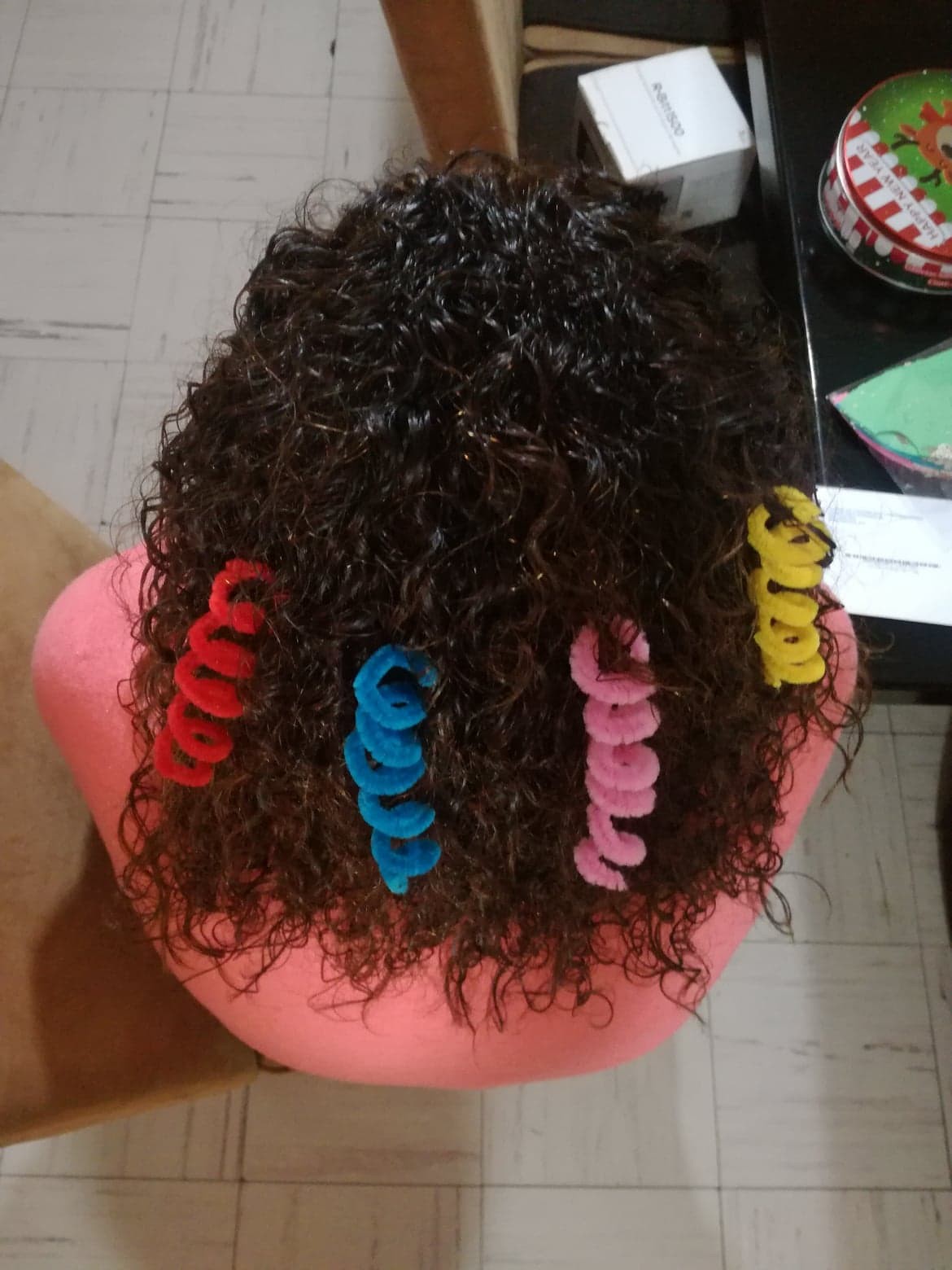In an indoor setting, a top-down photograph captures the back of a woman with dark brown, curly hair adorned with four brightly colored soft curlers: red, blue, pink, and yellow, from left to right. She is dressed in a pink outfit and positioned on a white, marble-mimicking tiled floor. To the top right of the image, a festive holiday tin with red and white stripes and a green top featuring a reindeer and the words "Happy New Year" adds a seasonal touch.